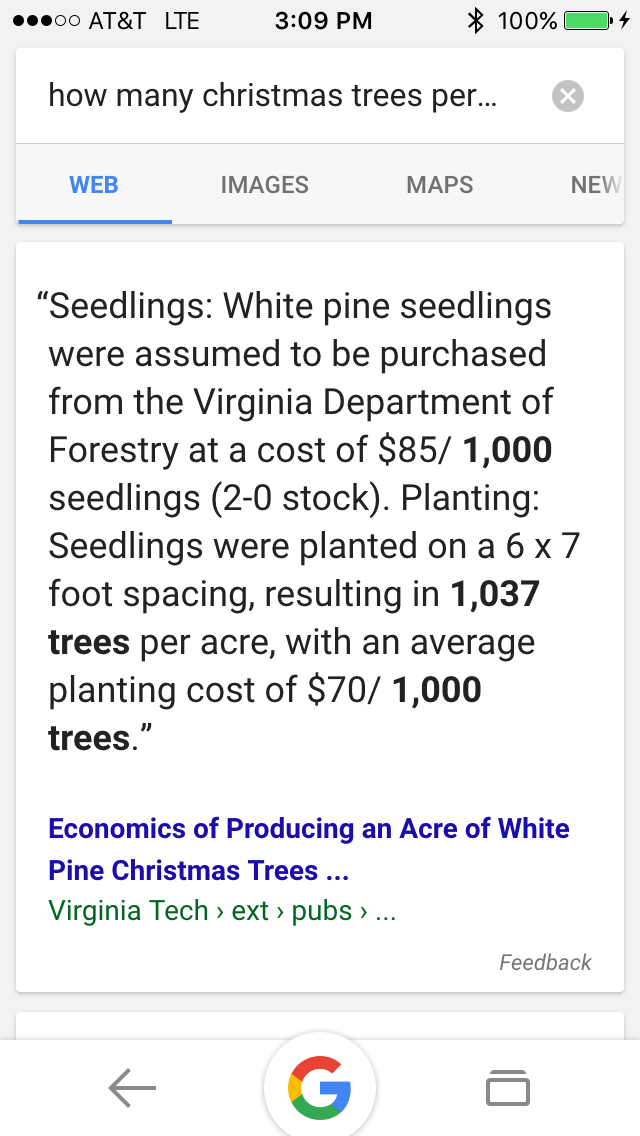This is a detailed screenshot of a smartphone displaying a webpage from Google under the AT&T LTE network, with three signal bars, the time at 3:09 PM centered at the top, and a fully charged battery icon in green. The search bar at the top contains the query "how many Christmas trees per," followed by menu options for 'Web' (highlighted), 'Images,' and 'Maps' in a dark text. The main content includes a description: "Seedlings. White pine seedlings were assumed to be purchased from the Virginia Department of Forestry at a cost of $85 per 1,000 seedlings (2-0 stock). Planting: Seedlings were planted on a 6 by 7 foot spacing, resulting in 1,037 trees per acre with an average planting cost of $70 per 1,000 trees." Under this text, a blue link reads "The Economics of Producing an Acre of White Pine Christmas Trees," referencing Virginia Tech Extension publications. The screen also shows the Google insignia, a left-pointing arrow, and a downward-pointing rectangle icon at the bottom, indicating navigation options.